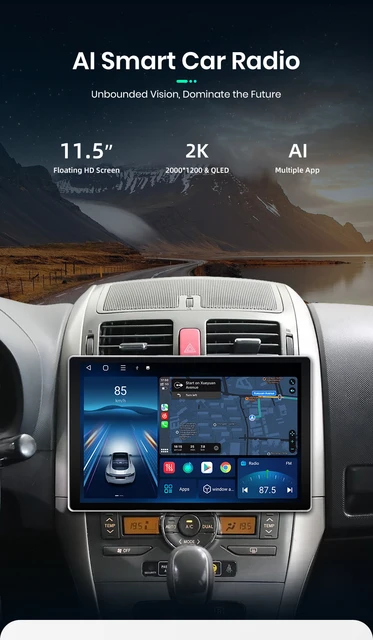This vertical image, resembling an ad, showcases the interior of a car, specifically focusing on the dashboard. Prominently displayed at the top center is the text "AI Smart Car Radio," followed by the line "Undaunted Vision, Dominate the Future." Below, three distinct text features appear: "11.5 inches floating HD screen," "2K, 2000 x 1200, QLED," and "AI Multiple App." The central focus of the image is a sleek, tablet-like 11.5-inch floating HD screen positioned in the middle of the dashboard. This advanced AI smart car radio screen displays various functionalities, including apps, radio, directions, and real-time speed. Additional features visible on the dashboard include AC controls, seat warmers, defrosters, warning lights, and flashers. The screen also shows a map, the current weather, and an image of the car on the road. Through the car's window, you can see a picturesque view of mountains and the road ahead, highlighting the state-of-the-art technology of this AI smart car radio.